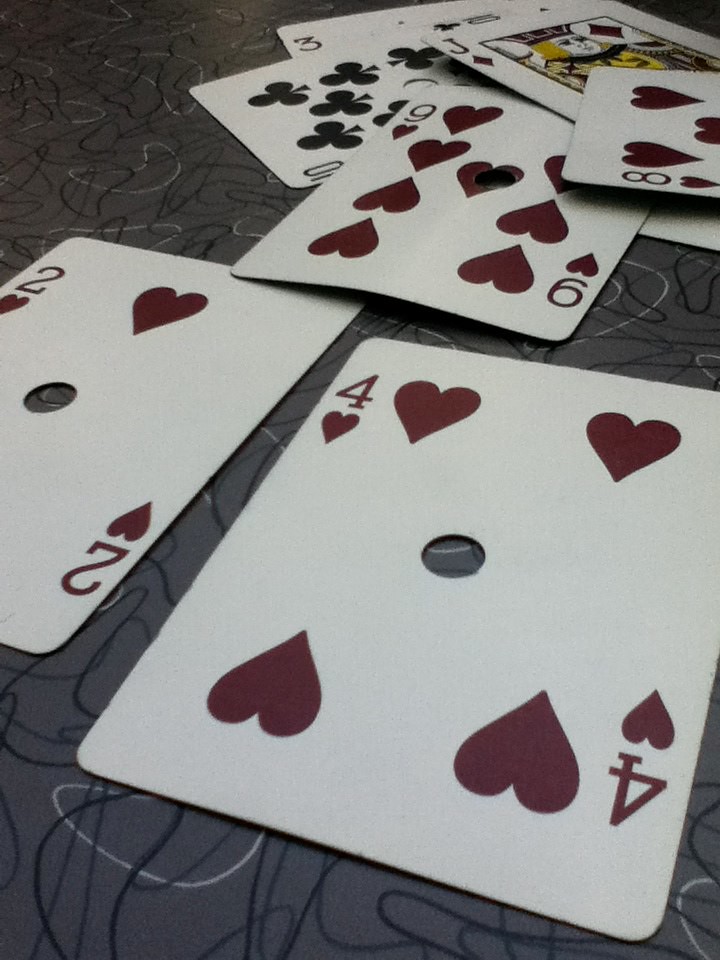A detailed photograph captures an array of unique playing cards spread across a gray, patterned carpet commonly found in medical or pediatric offices. The carpet itself features an abstract design composed of various black and white shapes. Central to the image is an extra-wide, nearly square playing card displaying the four of hearts, complete with four heart symbols and a distinctive hole punched through the center. Surrounding this focal card are other cards with similar designs, including the two of hearts, nine of hearts, eight of hearts, joker of diamonds, ten of spades, and partially visible three of clubs. Each card, consistent with the four of hearts, has a central hole and showcases a number of heart symbols corresponding to its value. The cards appear somewhat shuffled yet remain visually distinct against the intriguing backdrop.